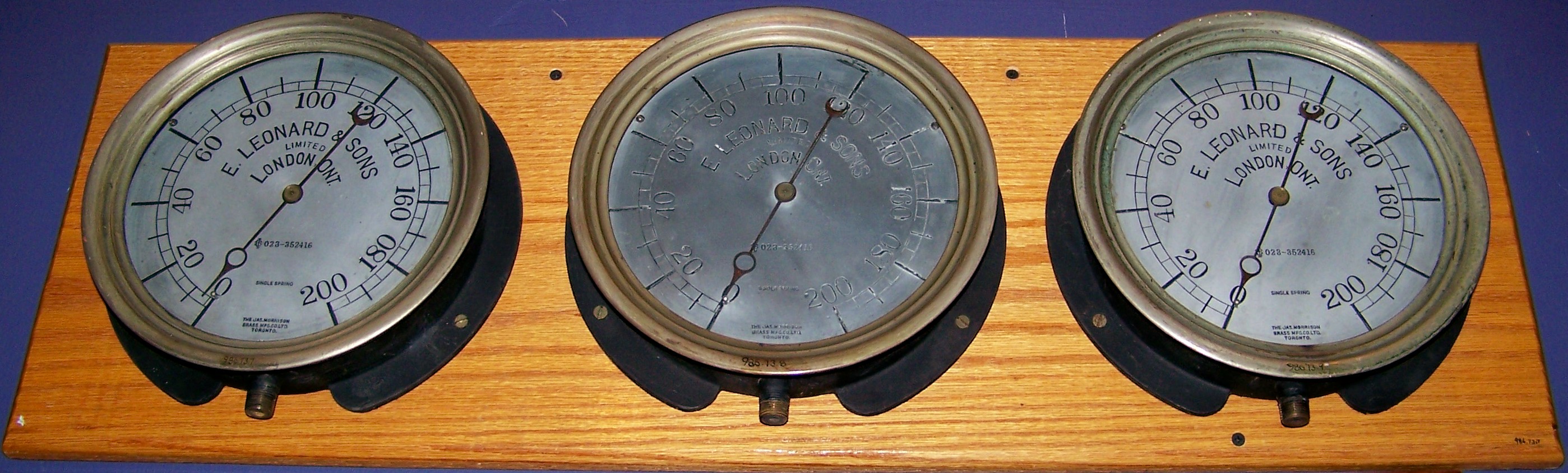The image showcases three vintage meters mounted on a basic beige piece of plywood. The meter on the left is clearly labeled "E. Leonard and Sons" and features a scale ranging from 0 to 200, suggesting it might be a speedometer. The central meter also has a scale up to 200, but its markings are less legible due to the absence of a clear faceplate, having only etched indentations. The meter on the right mirrors the one on the left in both design and scale. All three meters exhibit signs of wear, hinting at their age and frequent use. The background shows a hint of blue, possibly indicating the meters are placed on a blue tablecloth or surface. The overall appearance suggests that the image is a cropped section of a larger picture.